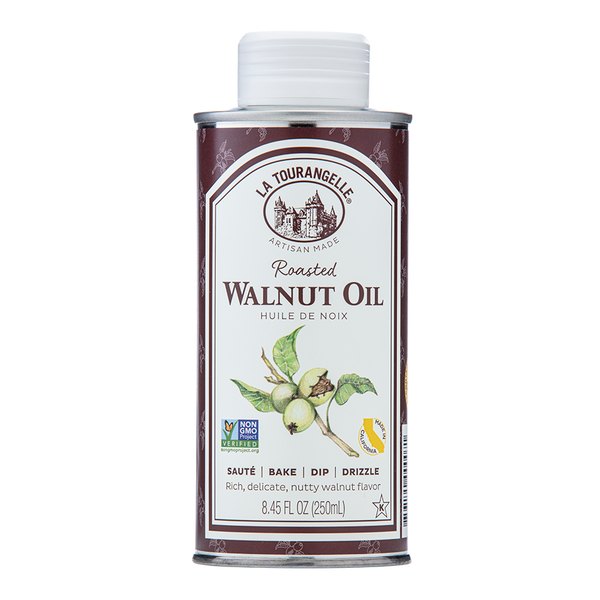The photo depicts a beautifully designed bottle of La Tourangelle Roasted Walnut Oil. The bottle, which has a purple hue and a white screw-on cap, features a brownish label with an elegant castle logo. Proudly stating "artisan made," the label emphasizes its rich, delicate, and nutty walnut flavor. Detailed images include part of a walnut tree, green leaves, walnuts, and an open walnut revealing its brown interior. The bottle is adorned with a "non-GMO" sign, verified by a butterfly project, indicating its high quality. It mentions versatile uses including sautéing, baking, dipping, and drizzling, and has a capacity of 8.45 fluid ounces (250 milliliters). This gourmet oil, imported from France, reflects exquisite attention to detail in both its presentation and its crafting.